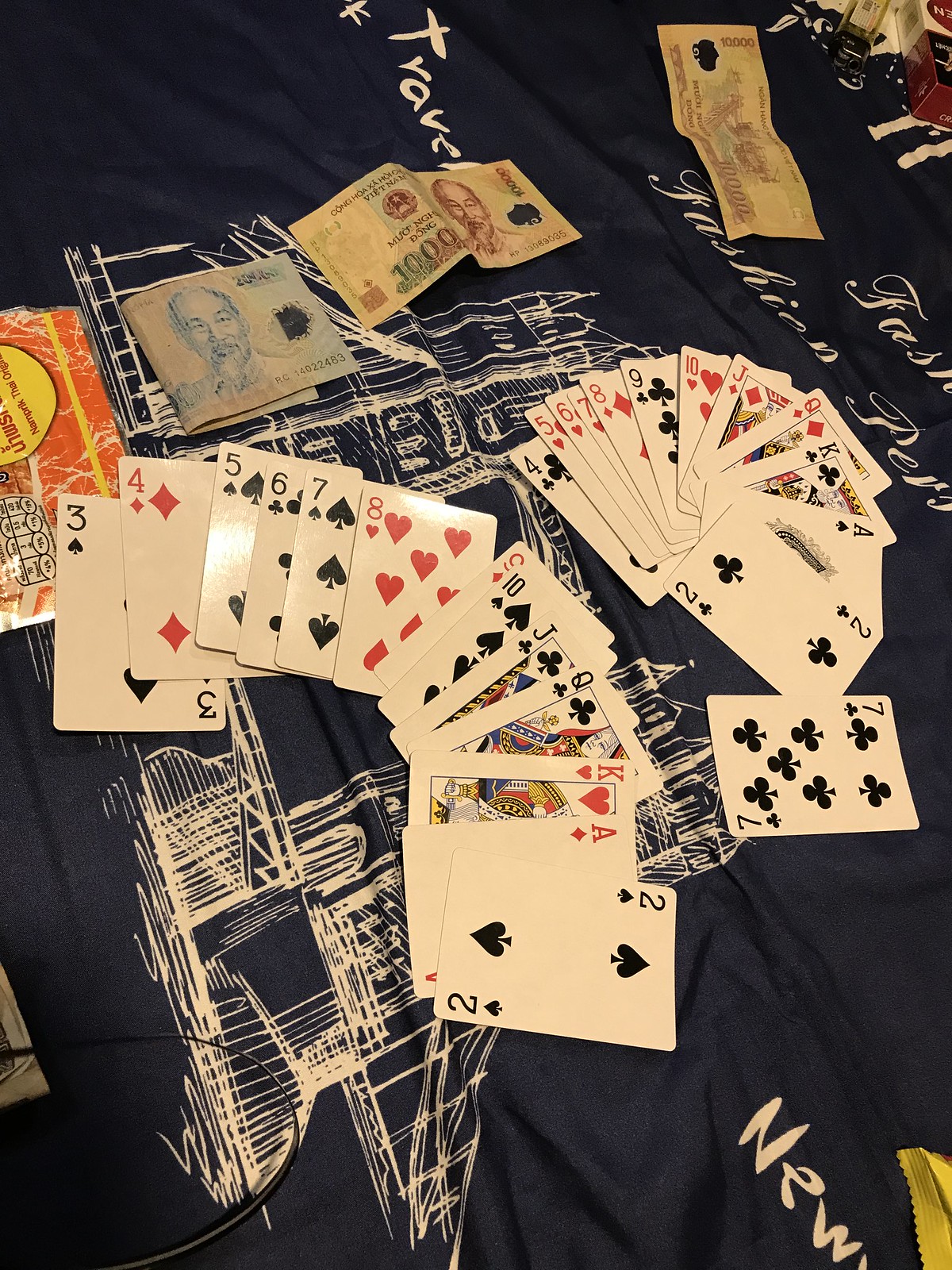Spread across a cloth printed with a partially obscured image of what appears to be the iconic Tower Bridge, complete with its twin towers, windowed structures, and suspension segments, is an array of playing cards organized into large hands. The cloth also features various partially legible texts including the words "NEW," "travel," "fashion," and an indecipherable acronym "PEV."

Among the cards lie three pieces of Vietnamese currency, adorned with the likeness of a bearded man in two different colors. The first bill, on the left, is folded and obscures much of its detail. The central bill, which is clearly a 1,000 dong note, displays the word "Vietnam" amid the surrounding Vietnamese text. The final, unfolded bill on the right is a 10,000 dong note, featuring what seems to be a landscape scene rather than a portrait. Each bill is marked by a distinctive die-cut feature, likely serving as a security measure.